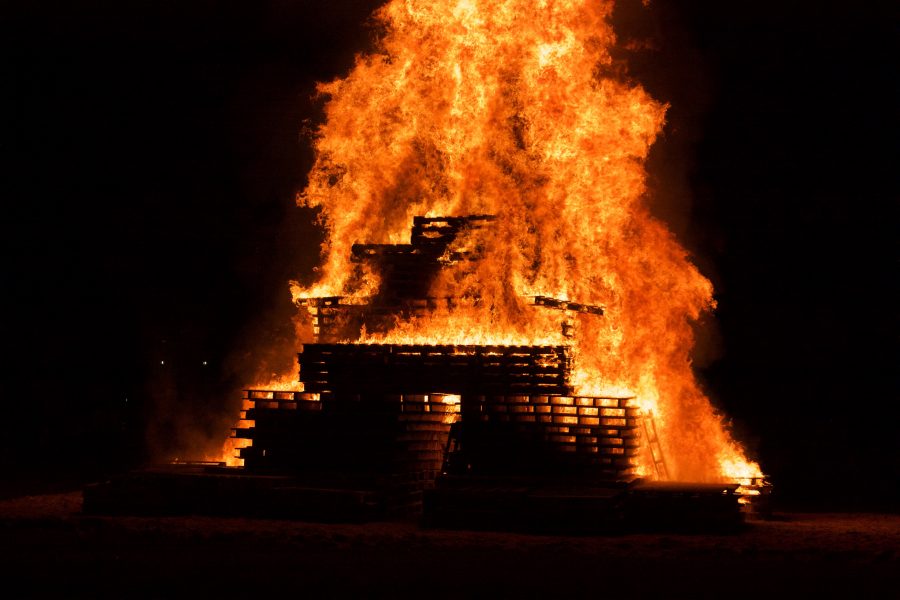This image captures a dramatic nighttime blaze consuming a towering stack of shipping pallets. The scene is predominantly dark, with concrete ground barely visible at the bottom, while the vivid, towering orange flames dominate the center, casting an intense light that illuminates the vicinity. The pallets are stacked in multiple tiers, high and tightly grouped, creating a massive inferno. While some remnants of the structure suggest it might have once been a building, the fierce flames obscure any clear identification, leaving charred wood and skeletal tiers as the main remnants. Smoke billows upwards, adding to the chaotic scene. Notably, there are no people or vehicles visible, implying the fire is left to burn itself out, its magnitude and brightness stark against the surrounding darkness.